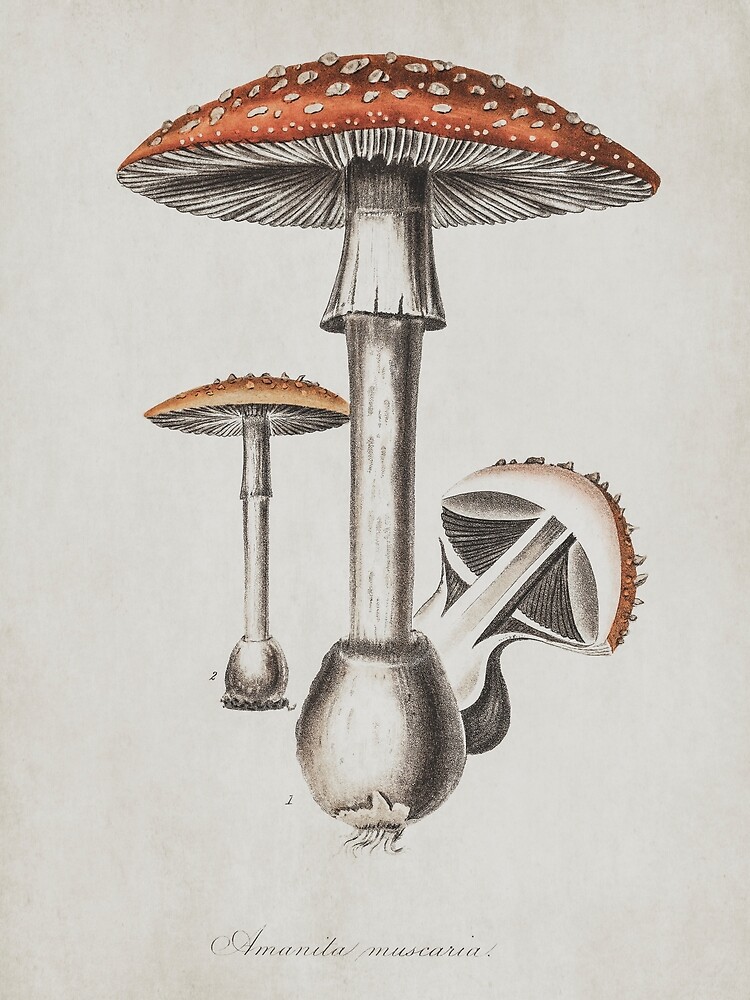This illustration portrays a detailed, hand-drawn, and colored scientific depiction of the Amanita muscaria mushroom, also known as the Santa Claus mushroom. The image predominantly features three mushrooms set against an off-white, slightly grayish background, giving it an aged, educational appearance. Each mushroom displays the characteristic red cap adorned with white spots, white stems, and distinctive white bulbs at the base. One mushroom is sliced in half, revealing the intricate white gills and internal structures for educational purposes, with parts labeled by numbers. At the bottom of the illustration, the Latin name "Amanita muscaria" is clearly inscribed. The drawing maintains a mellow tone while presenting a slightly three-dimensional and realistic portrayal of the mushrooms, emphasizing its scientific and educational intent.